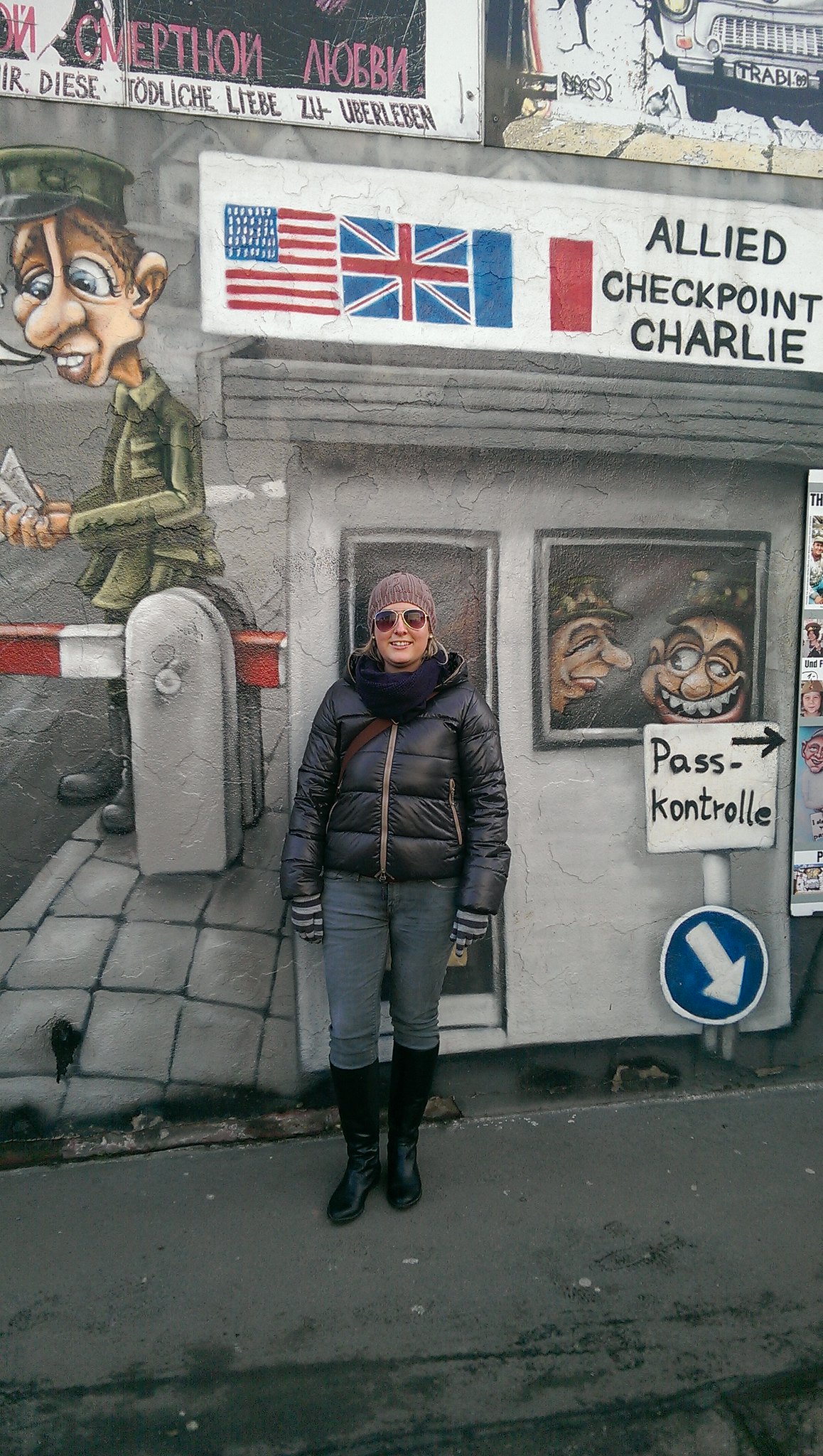A woman stands on a black asphalt street in front of a detailed mural, painted on a concrete wall, that depicts an Allied military checkpoint. The woman, who is Caucasian, is dressed warmly in a big black jacket, blue jeans, and high black boots. She accessorizes her outfit with a stocking cap and aviator sunglasses, and she has a bag strapped across her body. The mural itself is predominantly gray and illustrates a guard shack labeled "Allied Checkpoint Charlie" with American, British, and French flags above it. The guard shack features caricatures of military personnel in the windows with exaggerated, goofy expressions. To the left of the mural, there is a red and white control point gate and a large caricature of a soldier standing guard. Additionally, a sign below the soldiers in the shack reads "Pass Control" with an arrow pointing to the right, indicating directions at the checkpoint. The intricate and vibrant street art provides a striking backdrop for the scene.